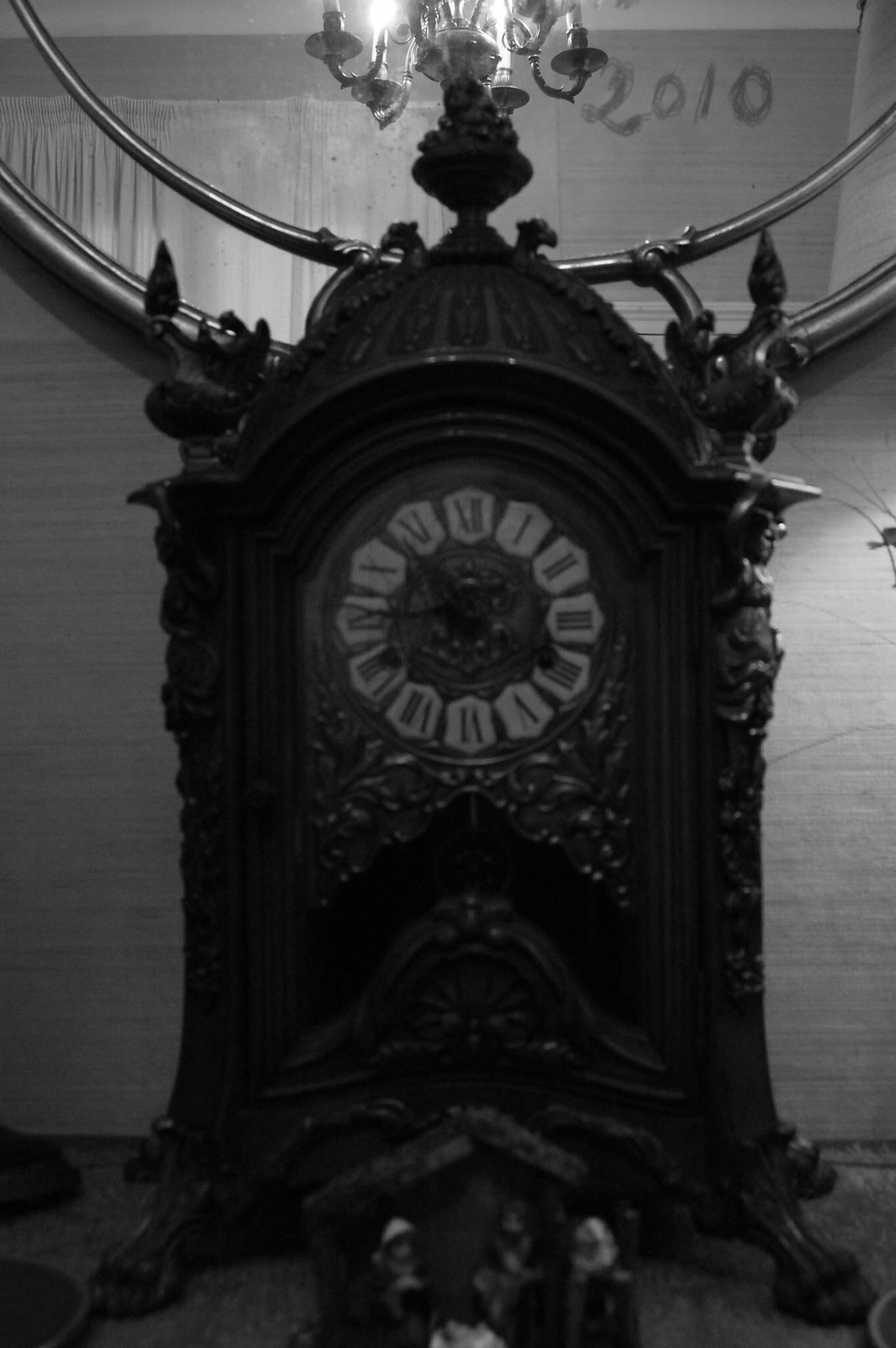The black-and-white image captures an ornately designed antique clock reminiscent of vintage cuckoo clocks, featuring a gothic aesthetic. The clock stands on intricate claw feet, and multiple figurines adorn its structure, contributing to its eerie, timeless aura. Notably, a significant figurine positioned in front of the clock evokes the Nativity scene within a chapel. Behind the clock, a mirror with dual concentric gold circles reflects part of the room, including a chandelier that adds to the overall dramatic effect. Faintly visible in the dust on the mirror is the year "2010," hinting at a long period of neglect. The photograph's dark tones and detailed elements enhance its haunting, antique ambiance.